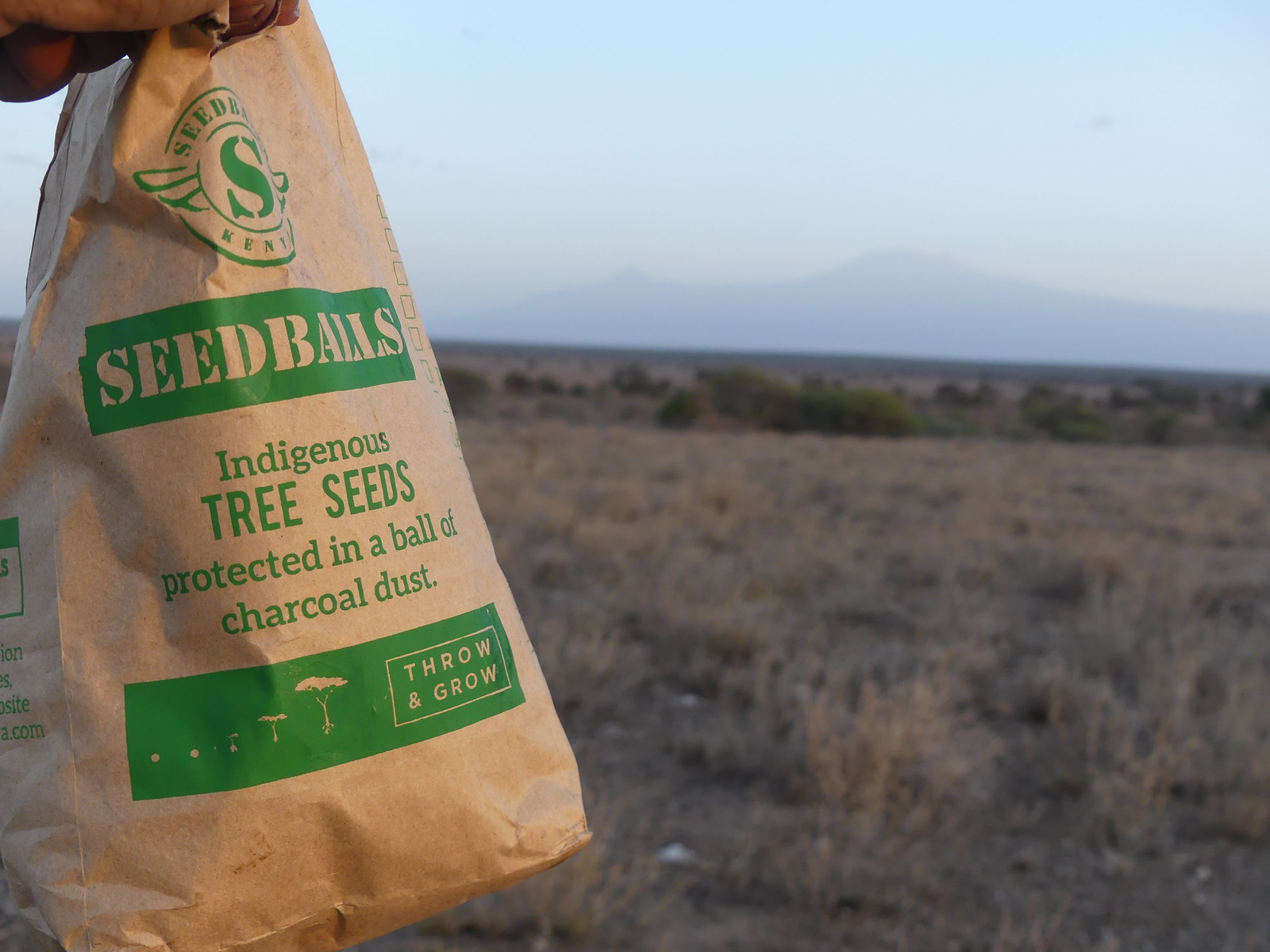The photograph captures an outdoor scene in what appears to be a large field, possibly near dawn or dusk. The ground is covered with dry, tan grass of varying lengths, interspersed with some green plants. In the distance, there is a faintly visible hilly or mountain range, tinged blue and blurred due to the depth of field, set against a nearly cloudless blue sky. 

On the left side of the image, a hand is prominently holding a brown paper bag adorned with green text in different fonts and styles. The text reads, "Seed balls, indigenous tree seeds protected in a ball of charcoal dust, throw and grow." The phrase "tree seeds" is in all caps, and "seed balls" appears in a stencil-like font within a green rectangle. The bag is approximately the size of a lunch bag and appears quite full, suggesting it contains multiple seed balls, ready to be scattered to promote the growth of indigenous trees in the area.